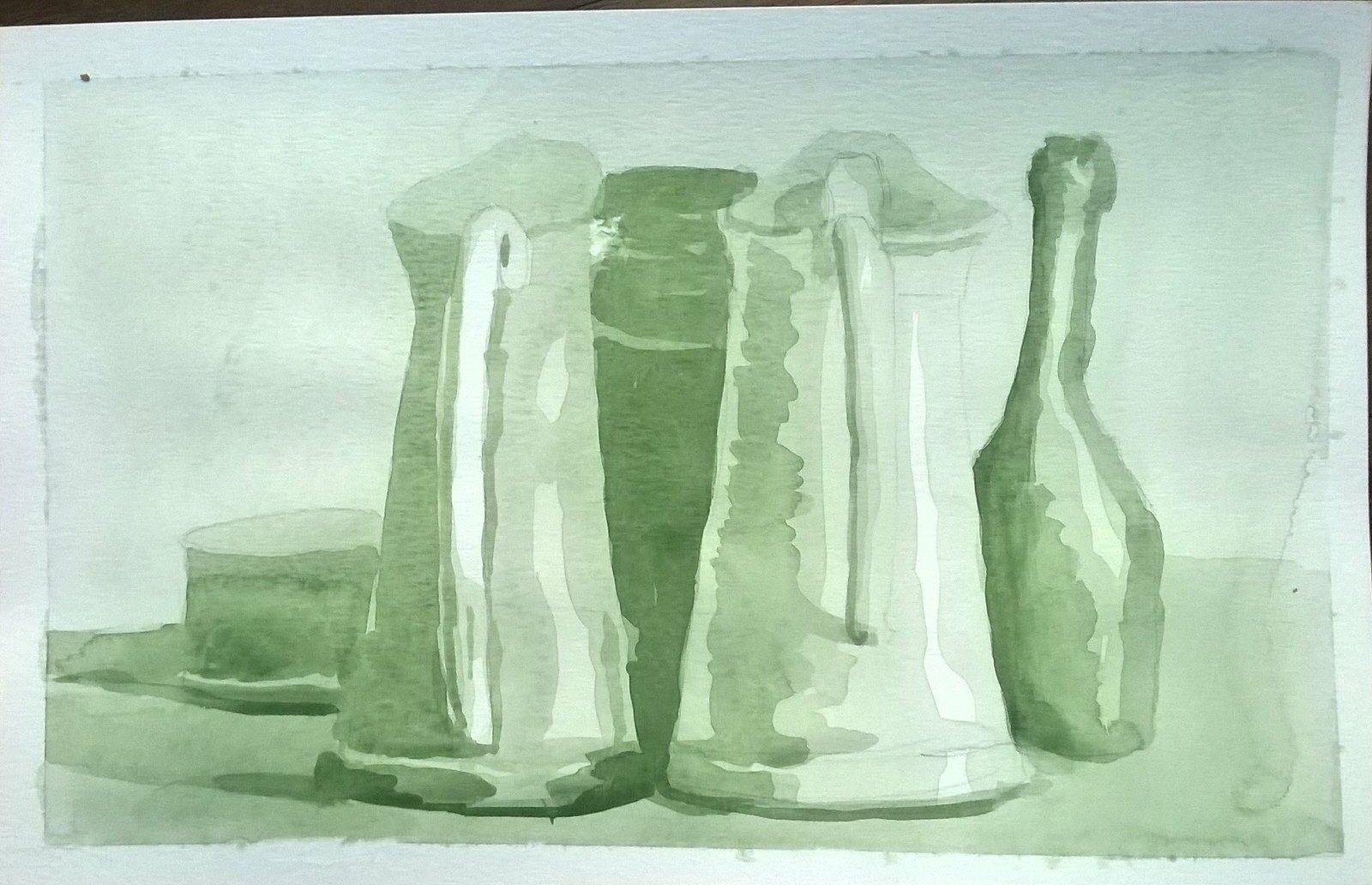The image depicts a serene still life rendered in a soft palette of pastel greens, ranging from pale grey-green to sage and light green. Dominating the composition are two large jugs, their handles oriented forwards, while the spouts point away. The light source emanates from the left, casting gentle shadows to the right of the primary jug, which reveals a rich texture suggestive of careful shading.

Nestled between these jugs is an ambiguous, dark green object, whose form is indistinct, leaving its identity open to interpretation—perhaps another jug or a unique container. On the far left, a smaller tub echoes the green tones of the jugs, enhancing the harmonious color scheme of the drawing.

Completing the scene on the right side is a distinctively shaped wine bottle, likely handcrafted pottery, with its unconventional design adding an element of intrigue. The entire composition bathes in a tranquil ambiance, with the subtle interplay of light and shadow accentuating the delicate artistry of the drawing.